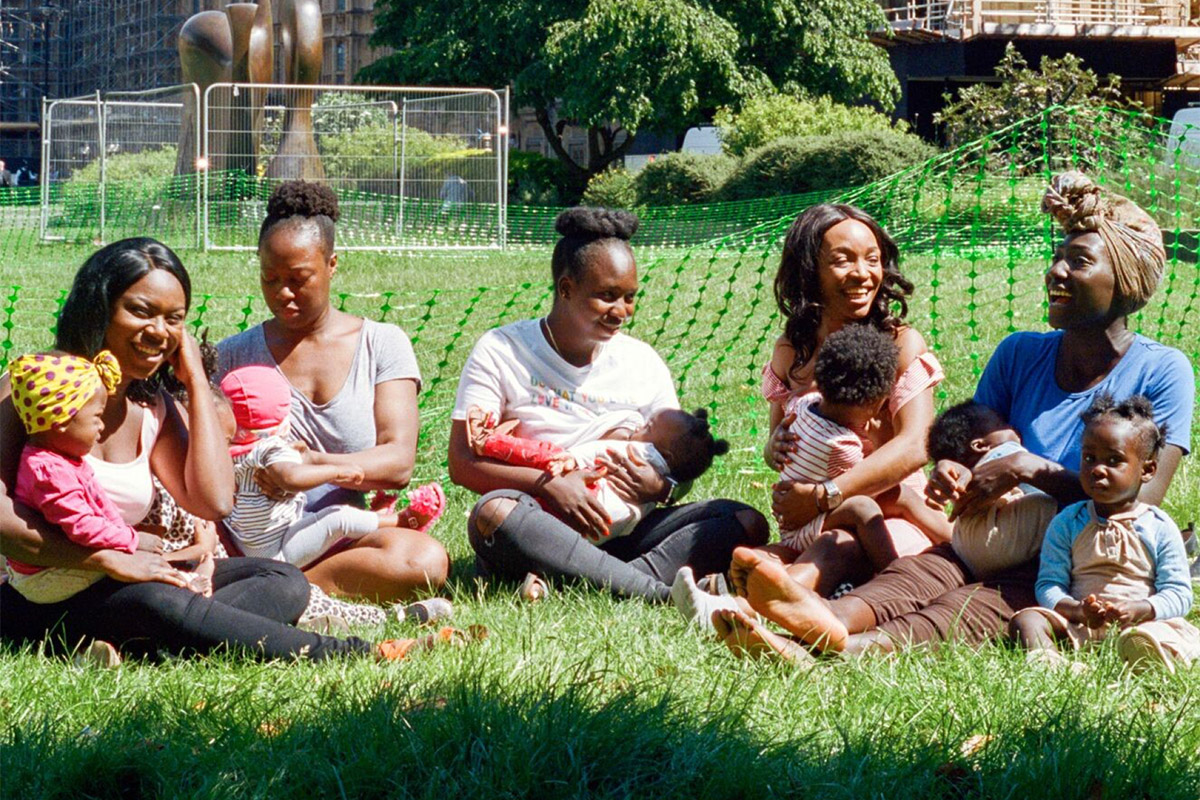This photograph captures a lively outdoor scene featuring five African-American mothers, each with their little children, seated on a grassy field in what appears to be a park. The day is bright and sunny, indicative of late spring or summer, with lush, fully-leaved trees and bushes providing a verdant backdrop. The mothers are arranged in a line, three on the left dressed in light-colored shirts, and two on the right, with one notably wearing a blue t-shirt and a head covering. She also has her legs outstretched and is surrounded by two children—a toddler close by and a baby on her lap, who may be nursing. 

To the left, a mother cradles a baby girl in a pink shirt and yellow head covering. Another mother with a pink head covering sits beside her, and the one in the middle sports pink pants. The child on the far right wears a striped shirt. The photograph, rectangular with the longer edges on the top and bottom, captures additional elements in the background: a temporary metal fence encircles a brass sculpture, and beyond that, there's a bent green plastic fence hinting at ongoing construction work. Further off, the scene includes towering high-rise apartments and other structures, blending urban elements with the serene park setting.